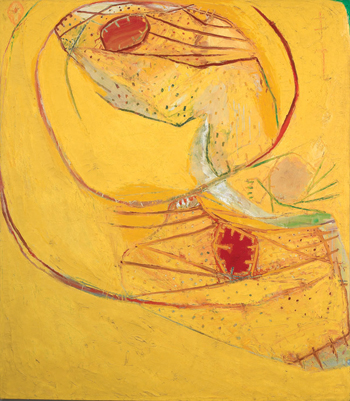The image depicts an abstract drawing characterized by a vibrant background in varying shades of yellow, ranging from mustard and golden tones to lighter, almost grayish hues. The most prominent feature is a red, donut-shaped line that curves around the upper center, resembling an imperfect circle drawn hastily. Within this circle, there are a few irregular, circular areas in red, accompanied by some subtle green specks. In the upper right-hand corner, a small patch of green appears as if it has stained the area. Below the red circle, towards the bottom right, there is a structure composed of horizontal and slightly slanted lines, with four lines protruding from it, and a touch of blue nearby. Additional green stripes and occasional white outlines further enhance the abstract nature of this artistic piece. While interpretations may vary, some viewers might see imagery like a snake's head with a red eye and green markings, or a rock with a crowned face that appears to be yelling.